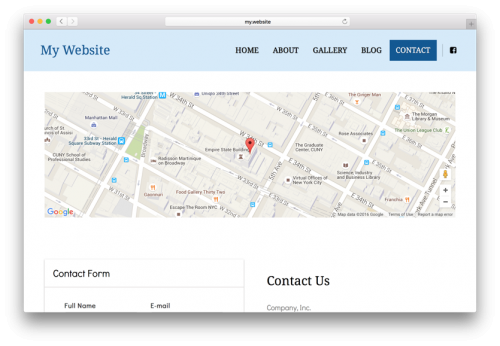This image captures a computer screen displaying a webpage titled "My Website," prominently presented in a blue font on a blue background stretching across the top of the page. Below this header, the navigation menu is displayed, featuring black text links for 'Home,' 'About,' 'Gallery,' and 'Blog,' alongside a deep grayish-blue button marked 'Contact.'

In the central section of the webpage, there is an embedded map, centered around a pinpoint marking the location of the Empire State Building. The map also shows street names, such as East 34th Street, providing context to the location highlighted.

Towards the bottom of the image, a contact form is visible, requesting a user's full name and email address. The form includes a prominent 'Contact Us' button and is labeled underneath with "Company Incorporated." The lower portion of the contact form and any additional details beyond this are cut off from view in the image.